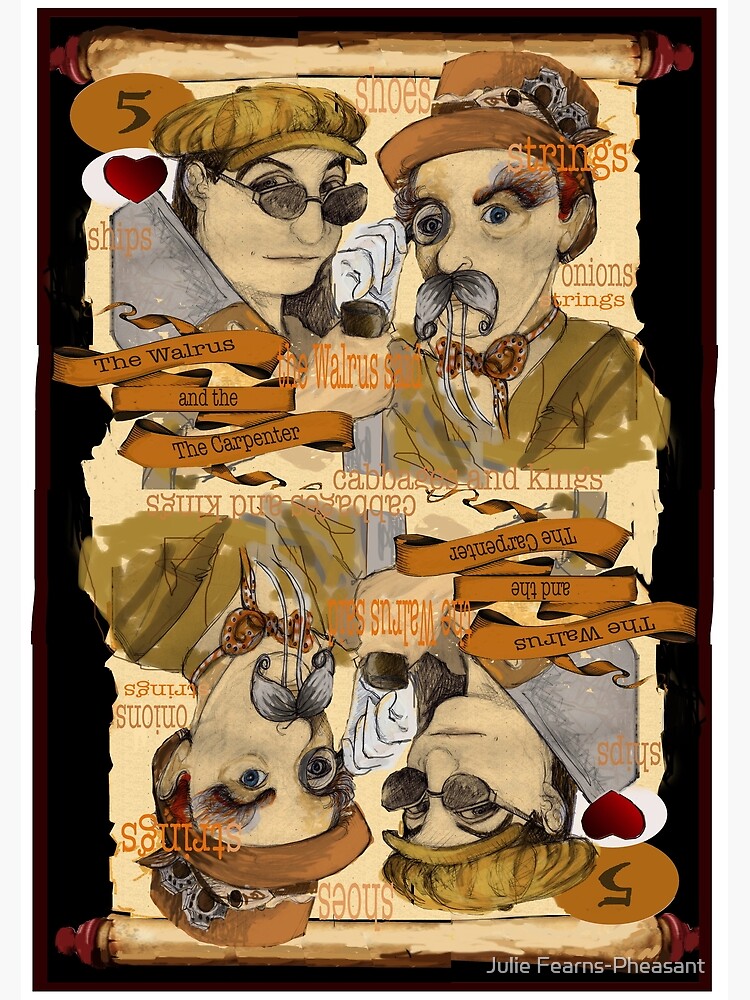This poster, styled in steampunk fashion, features a detailed and symmetric depiction of characters from a steampunk version of "Alice in Wonderland," specifically "The Walrus and The Carpenter." Presented in a portrait orientation, the background resembles a painted scroll with a red border surrounding a black center, giving it an antique look. The visual centerpiece is a paper-like scroll wound around wooden rods at both ends, reminiscent of a vintage banner.

In the top half, a number five in an orange circle and a red heart in a white circle are noticeable on the top left. Next to these symbols stands a woman, hand-painted, wearing dark sunglasses or possibly welding glasses, and an old-fashioned hat. Directly to her right is a man, also hand-painted, dressed in a suit and bowtie. He sports a monocle held up to his eye by a white-gloved hand, a downward curly mustache, wild eyebrows, and an orangish hat. This imagery is mirrored exactly in the bottom half, both horizontally and vertically, maintaining a perfect symmetric or reflected image.

Encircling the characters are various words associated with the original poem, such as "shoes, strings, ships, onions, cabbage, and kings," all subtly integrated into the design. The colors used in the artwork include tans, browns, whites, reds, and hints of orange, giving it an earthy and rustic palette. At the bottom right-hand corner, the artist's name, Julie Fearns-Pheasant, is inscribed in white. The whole visual composition is bordered by thematic banners proclaiming "The Walrus and The Carpenter," which contribute to the steampunk essence of the piece.